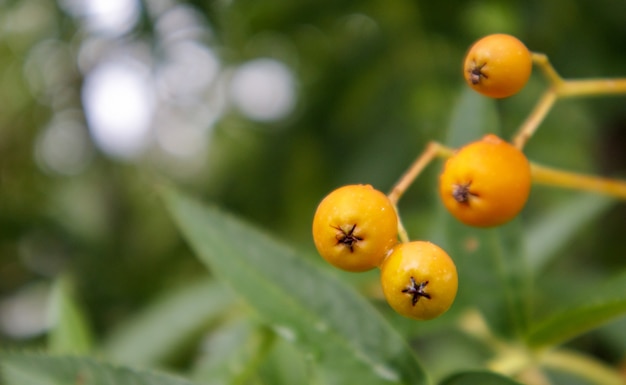This is a close-up photograph of a small cluster of four vibrant berries, yellow-orange in color, resting on a beige-brown stem. The berries, with their smooth surfaces, are the focal point of the image, drawing attention with their vivid hues. The photograph was taken outdoors during daylight, and in the softly blurred background, the impression of green leaves creates a lush natural setting. Delicate beams of light filter through the foliage, adding a touch of warmth and highlighting the natural beauty of the scene. No text overlays the image, allowing the viewer's focus to remain solely on the striking detail and serene ambiance of the plant.